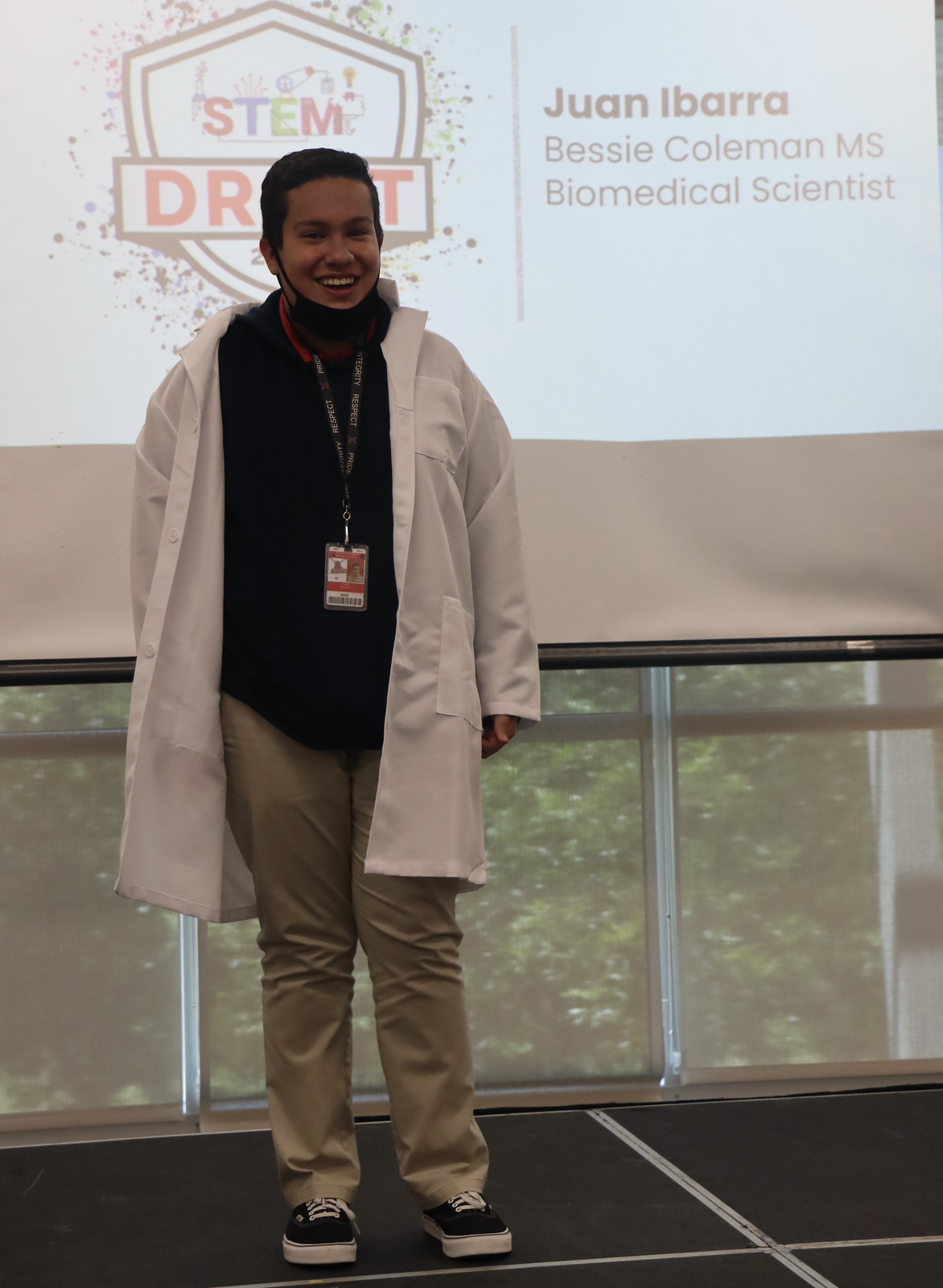This image features a young male named Juan Ibarra, who is a biomedical scientist associated with Bessie Coleman Middle School and a student of the STEM program. Juan is standing confidently in front of a presentation screen, likely delivering a talk. He is dressed in a white lab coat over a black top and khaki pants, with tennis shoes for comfort. An ID badge, indicative of either his school or the STEM program, hangs on a lanyard around his neck. Notably, he is also wearing a mask, though it is lowered, suggesting the photo was taken during the COVID-19 timeframe. He stands against a backdrop of tall glass windows, through which daylight reveals an outdoor scene with trees, indicating he is likely on the second floor of the building. Behind him, a display referencing STEM adds context to his academic focus and presentation. Juan has short, dark hair and presents a pleasant demeanor.